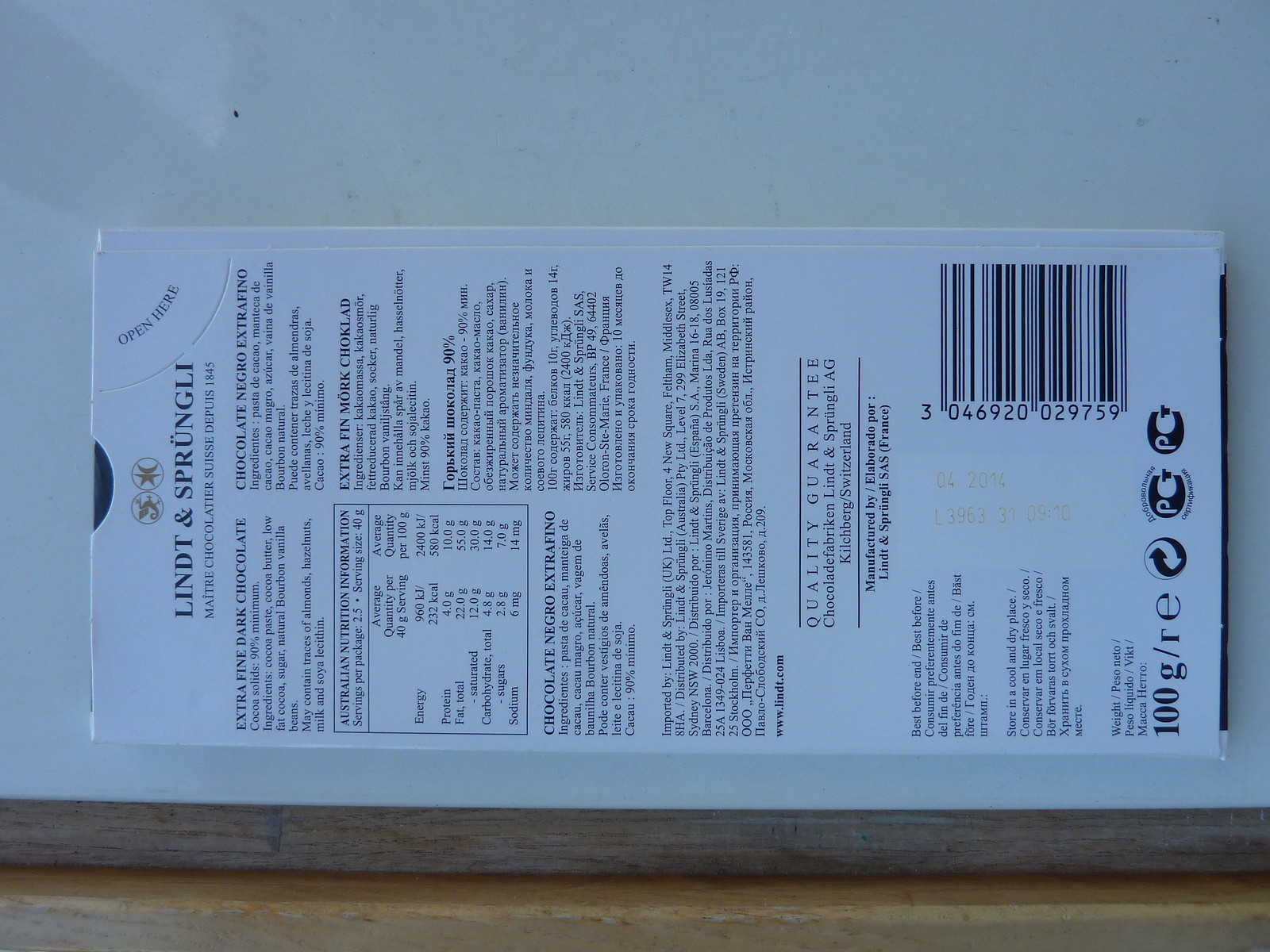The photograph captures the back of a 100-gram Lindt chocolate bar, which is placed on a pristine white surface with a wooden border at the bottom. The chocolate bar is positioned sideways, with the top of the package facing left and the bottom right. Dominating the top left corner is the barcode. The packaging provides information in multiple languages, including English, Spanish, Portuguese, Russian, and possibly Swedish, suggesting a diverse international audience. The nutritional facts, labeled as Australian nutrition information, imply that this particular bar originated from Australia. The detailed visual and textual elements on the packaging offer a comprehensive insight into the product’s origins and ingredients.